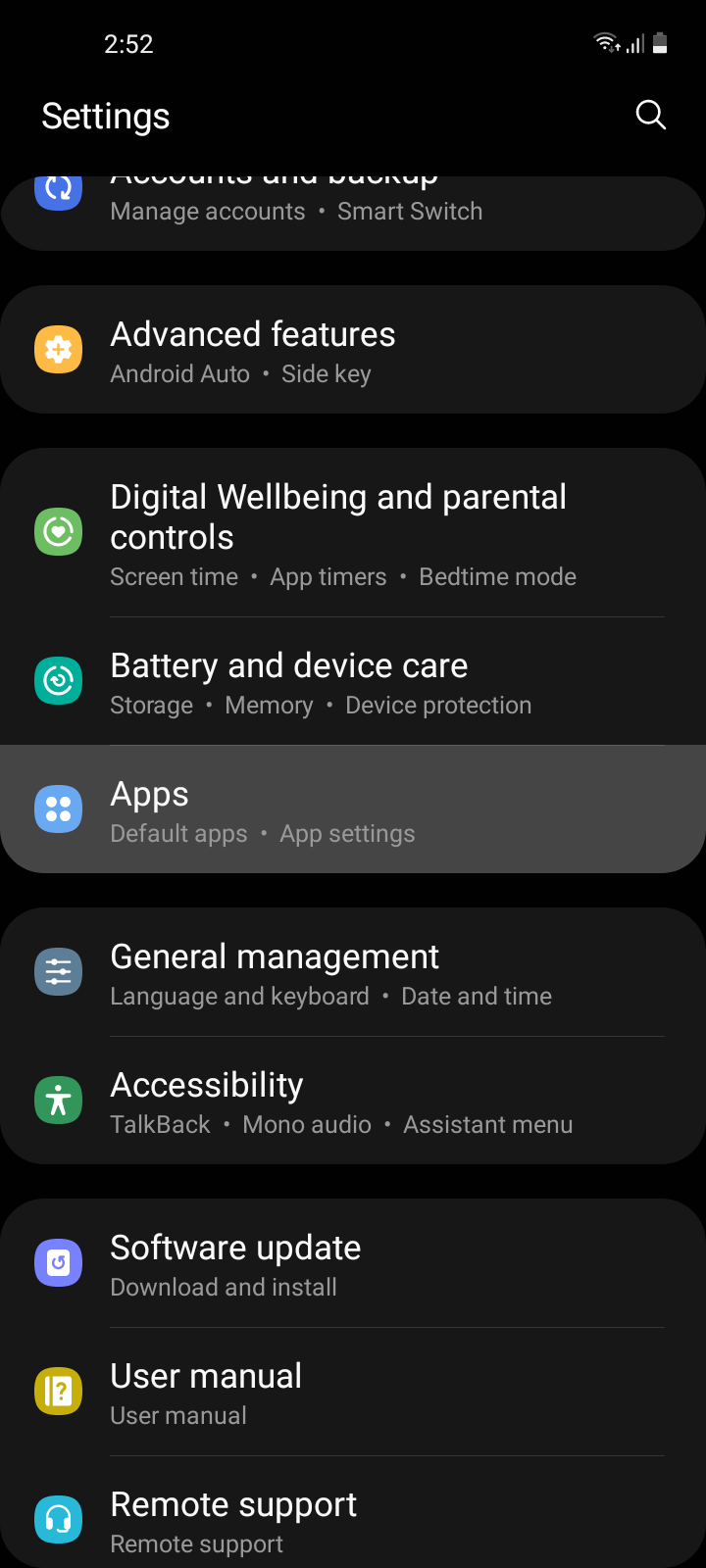This image is a detailed screenshot of a phone's settings screen with a predominantly black background and several gray tabs horizontally aligned. At the top left corner, approximately one inch from the edge, the screen displays the time "2:52" in bold white text. On the top right corner, there is a battery icon, half-filled with the top half in white and the bottom half in gray. Adjacent to it are the connectivity icons: three out of four white bars for cellular signal and three out of four white bars for Wi-Fi signal.

Directly beneath the time display, the word "Settings" is prominently shown in bold white text. On the top right next to "Settings," there is a search icon. Below this header is a thin gray border, beneath which a blue icon can be seen on the far left side, accompanied by partially visible text hinting at the "Accounts and Backup" section. Smaller gray lettering under this title reads "Manage accounts" and "Samsung Smart Switch."

Following this, there is a sequence of sections separated by black borders. The first section includes an orange square icon for "Advanced Features" with additional information beneath it. 

The next section has three icons vertically aligned and labeled: 
1. "Digital Wellbeing and Parental Controls" with three tappable options underneath.
2. "Battery and Device Care," also with three tappable options.
3. "Apps," highlighted in gray indicating it has been selected, showing "Default apps" and "App settings" below.

Another gray tab follows with two icons:
1. "General Management" with two tappable options.
2. "Accessibility" with three tappable options.

Below this, separated by another black space, there are three more gray tabs:
1. "Software Update" with one tappable option.
2. "User Manual" with one tappable option.
3. "Remote Support," also with one tappable option and an icon to the left.

The screenshot provides a clear and systematic view of the phone's settings, highlighting various sections and options available for user configuration.